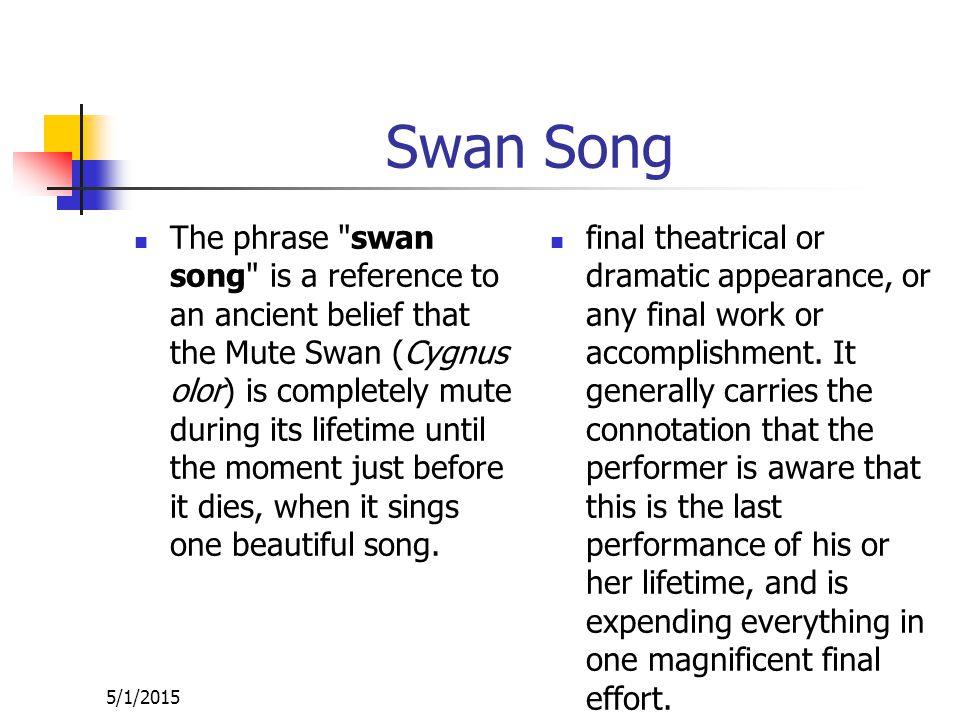The image is a slide with a white background, seemingly part of a PowerPoint presentation, dedicated to explaining the concept of a swan song. At the top of the slide, in blue letters, the headline reads "Swan Song." In the upper left corner, there is a logo consisting of three squares in yellow, red, and blue.

Below the headline, there are two bullet points, side by side. The left bullet point explains that the phrase "swan song" refers to an ancient belief that the mute swan (Cygnus olor) remains silent throughout its life until the moment just before it dies, when it sings one beautiful song. The right bullet point elaborates that a "swan song" denotes a final theatrical or dramatic appearance, or any final work or accomplishment, suggesting that the performer is aware this is their ultimate performance and is giving their all in a magnificent final effort.

Finally, at the bottom left corner of the slide, the date "5-1-2015" is displayed. The slide uses a combination of purple, black, white, yellow, red, and blue colors, with a well-organized layout that emphasizes the text.